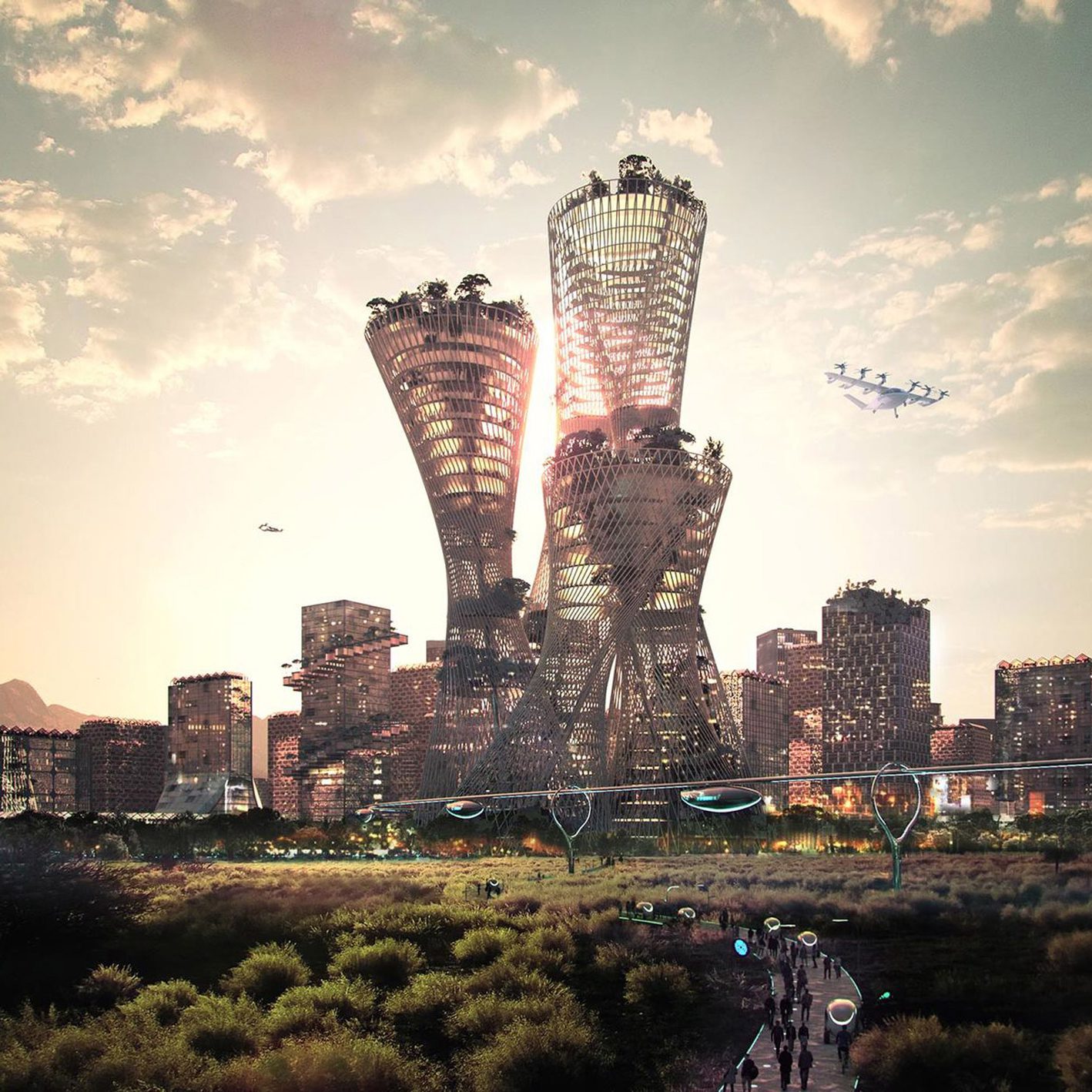This image presents a stunning, computer-generated depiction of a futuristic, potentially utopian cityscape at sunset. Dominating the frame are uniquely shaped skyscrapers, particularly three central, hourglass-structured towers adorned with lush greenery on their rooftops. Flanking them are additional skyscrapers, including a notable one with an external spiral staircase. Below, a well-lit, winding walkway snakes through a dense, park-like area bustling with people heading into and out of the city. A futuristic suspended railway hovers above, supported by structures reminiscent of metallic tennis rackets, with sleek train pods gliding towards the urban center. In the sky, an aircraft with extended wings featuring helicopter blades soars beside another mysterious flying object. The scene is bathed in the warm glow of the golden hour, highlighting the playful dance of light and shadow across the intricate cityscape.